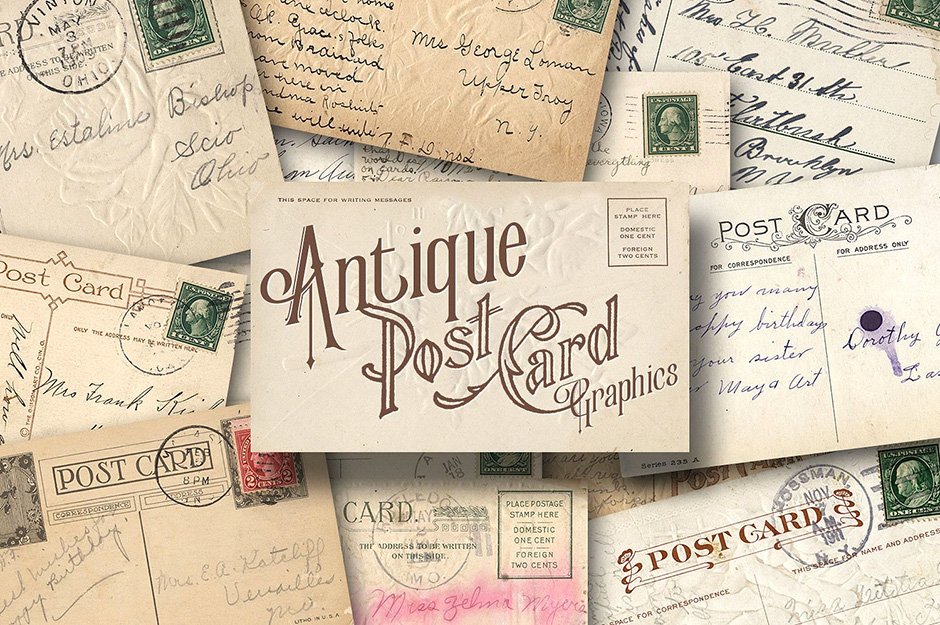The photograph depicts a vertically aligned collage of vintage postcards meticulously arranged, each turned to display the writing side. The focal point of the image is a centrally located postcard that reads "Antique Postcard Graphics," its text stylishly curved from the upper left to the lower right in a brown print. This central postcard also includes a small box in the upper right corner indicating "Place Stamp Here" with a cost of "Domestic one cent" and "Four and two cents," underscoring its antiquity.

Surrounding this main postcard are various other postcards exhibiting signs of age such as pink and brown stains. One notable postcard in the lower left corner bears a stamp resembling a dollar bill. Above the central card, another postcard is covered in cursive handwriting in blue ink, while to the right, a card exhibits a purple stain. Many of these postcards display typical old-time formatting where one side is designated for the correspondence and the other for the address. Several postcards also bear post office stamp marks, indicating they have been previously mailed. Managing to maintain an organized chaos, they appear to be stacked and layered at different angles, contributing to a rich tapestry of historical communication.